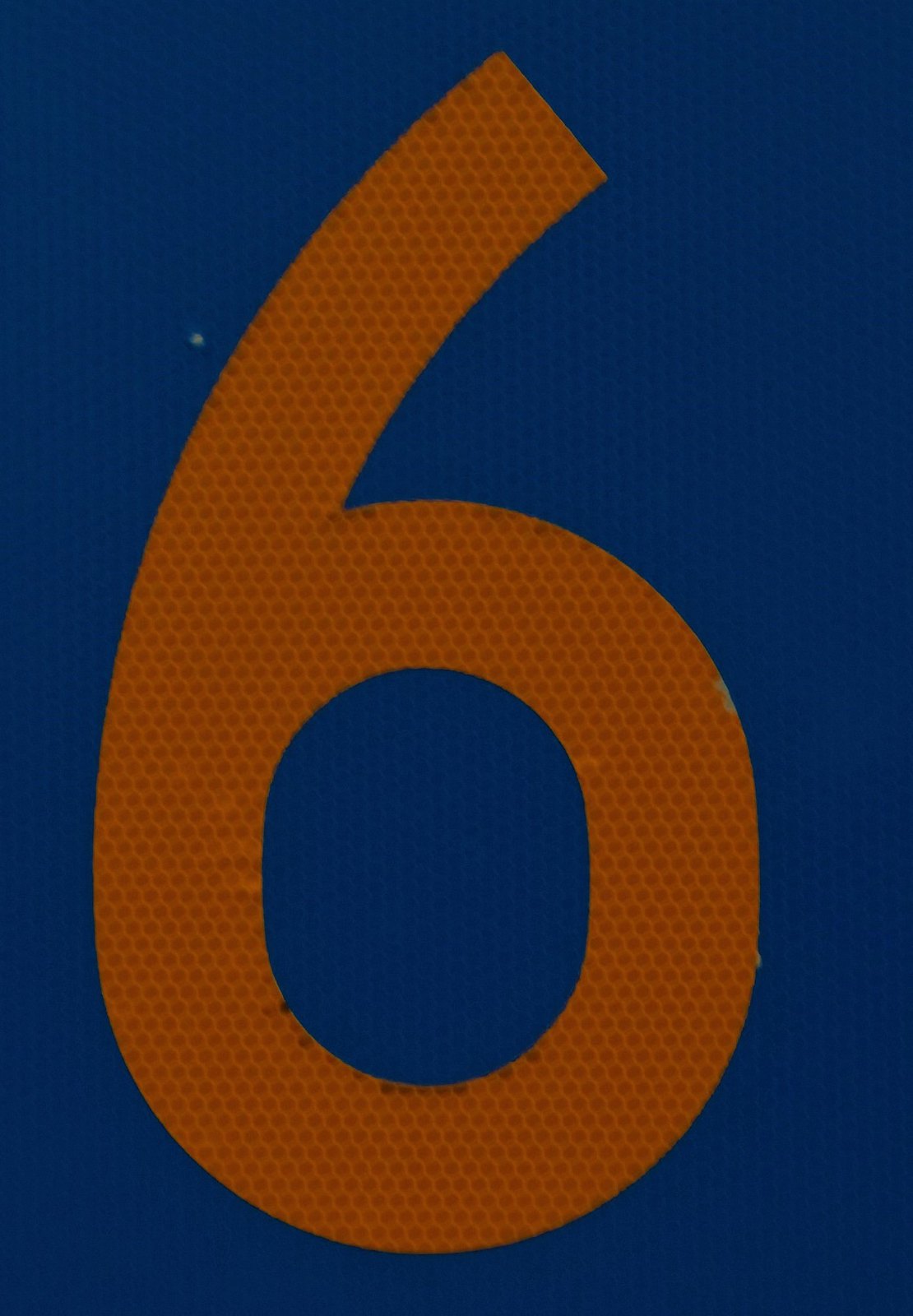The photograph features a striking, bright orange number six set against a royal blue background that resembles fabric, possibly from a jersey or shirt. The image, which is about twice as tall as it is wide, showcases the number six filling up most of the available space, leaving roughly 5% of the area at the top and bottom and 15-20% on the sides. The number six seems to be constructed from numerous tiny hexagons, with a lighter orange outlining the shapes and a darker orange filling them in, giving it a textured appearance reminiscent of a basketball. Notably, the inner loop of the six reveals patches where the fabric underneath has become visible due to the hexagons peeling away or lifting, particularly around the intersections and curves, creating small air tunnels. These details collectively suggest wear and tear, as if the number has begun to detach from its fabric base over time.